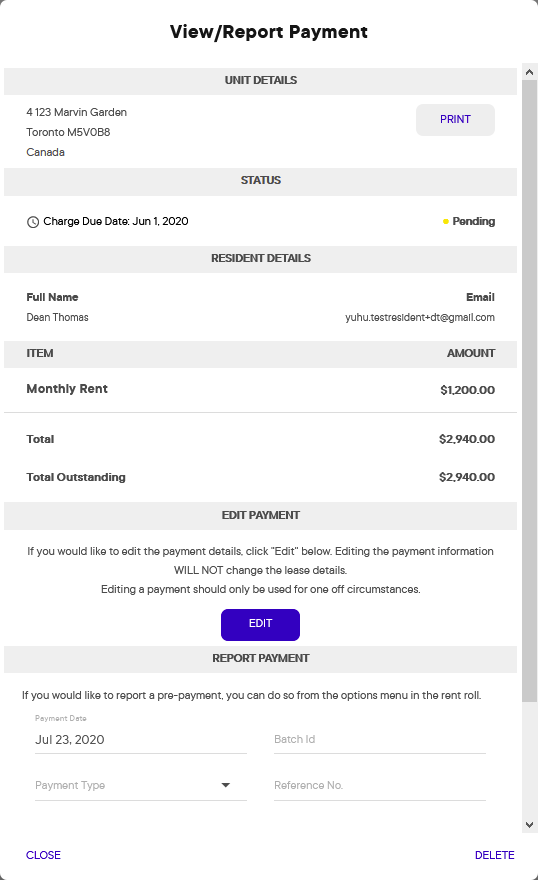This image is a detailed screenshot, shaped like a phone screen. At the top, bold black text reads "View / Report Payment." Beneath this, the interface shows several sections which can be navigated through a scroll bar that is currently positioned at the top.

The first visible section is a grey banner labeled "Unit Details" in a slightly darker grey font. Under this banner, the address "123 Marvin Garden, Toronto, Canada" is displayed. To the right of this address, there is a small tab labeled "Print."

The subsequent grey bar is titled "Status." Within this section, the information "Change Due Date: June 1st, 2020" is displayed with a status of "Pending" to the right.

Following this, the "Resident Details" section lists the full name "Dean Thomas." To the right, there is an email address provided under a subheading labeled "Email."

Another grey bar appears, marked "Item," which details the monthly rent amount as $1,200 CAD. Further, it states the "Total" as $2,940 and the "Total Outstanding" as $2,940.

Additionally, the screenshot includes an option labeled "Edit Payment" in blue, indicating that users can modify payment details by clicking the Edit button, though no edits have been made. It also presents a button labeled "Report Payment" for reporting a prepayment.

The date "July 23rd, 2020" is visible at the bottom of the screenshot, possibly indicating the last update or payment entry date.